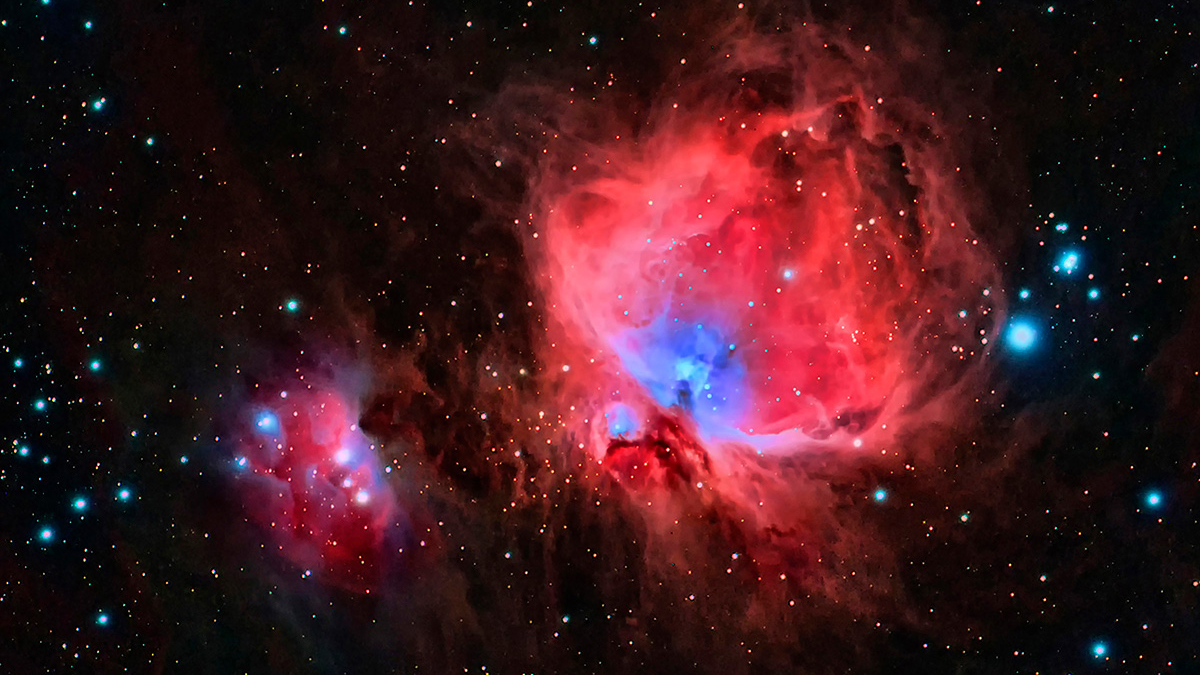This stunning landscape-oriented, high-definition image of outer space showcases a vast dark, black expanse dotted with numerous stars: some small and orange or yellow, while others are larger and blue. Dominating the center of the photograph is a brilliant and intense red cloud, reminiscent of a glowing fireball with smoky tendrils. This red nebula features areas of pink towards the top, transitioning into a deeper, vibrant red. Within this nebulous region, there are two main red cloud clusters, punctuated by dark gaps and glowing with neon blue light at their base and in the core. Smaller bright blue stars and round lights shimmer around the red cloud, adding contrast and depth. The image captures the splendor and mystery of a distant galaxy or constellation, making the fiery red nebula the focal point against the serene backdrop of the night sky.